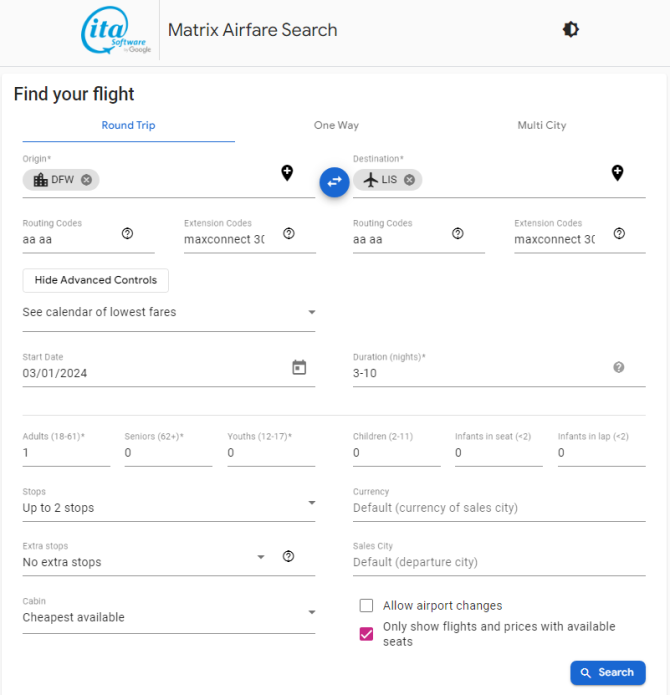The image showcases an airfare search interface for booking flights. At the top, the header displays logos for "ETA Software" and "Google," with "Matrix Airfare Search" prominently to the right. An icon featuring a sun, split into a half-black, half-white design, is also visible.

Below the header, the main search panel begins with several flight type options: "Round Trip," "One Way," and "Multi-City." The fields for specifying the journey show "Origin: DFW" and "Destination: LIS," separated by a plane icon.

Further down, there is a section for entering "Routing Codes," which lists: AA, AA, AA, and "Extension Code: MaxConnect 3." This is repeated again for routing code entries. There are options available to "Hide Advanced Controls" or view the "Calendar of Lowest Fares."

The search criteria includes a start date of "3-1-24" and a trip duration of "3-10 nights." Passenger details are specified as follows:
- Adults: 1 (aged 18-16)
- Seniors: 0
- Youths: 0
- Children (aged 2-11): 0
- Infants in seat (under 2 years): 0
- Infants in lap (under 2 months): 0 

Search preferences allow up to "2 stops" and the flight currency is set to the "Default currency of sales city." The search further specifies no extra stops, the "Default departure city" for the sales city, and the "Cheapest available" cabin class.

Additional options include checkboxes for allowing airport changes and showing only flights and prices with available seats, the latter of which is selected. This checkbox is highlighted with a purplish background and a white checkmark.

Finally, a prominent search button at the bottom right, blue with white text, invites users to commence their flight search.

The interface is set against a user-friendly, visually organized backdrop to facilitate efficient flight booking.